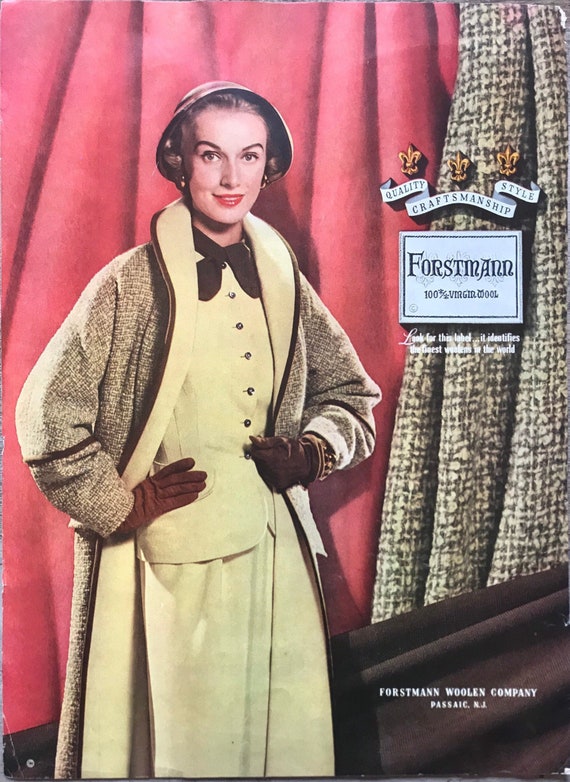The image is a vintage advertisement from the 1960s promoting a woman's coat. The background features a rich red curtain, adding a theatrical feel to the scene. In the foreground stands a sophisticated woman. She is adorned in a brown bucket hat and has her hair neatly tucked underneath. Her outfit includes a long tweed jacket with a brown and light yellow pattern on the outside and yellow on the inner lapels. She wears a matching dress suit, with a yellow buttoned top and yellow skirt underneath, complemented by a maroon-colored tie and gloves. The woman's poised smile is accentuated by her red lipstick and brown eyes.

On the right side of the poster, a white ribbon with black text reads, "Quality Style Craftsmanship." Directly below, the brand name "Forstmann" is prominent, within a black rectangle border, followed by the phrase "100% Virgin Wool." At the very bottom right corner, the text reads, "Forstmann Wool & Company, Passaic, New Jersey," over a brown background. The detailed fabrics and overall design emphasize the luxury and craftsmanship of the Forstmann brand.